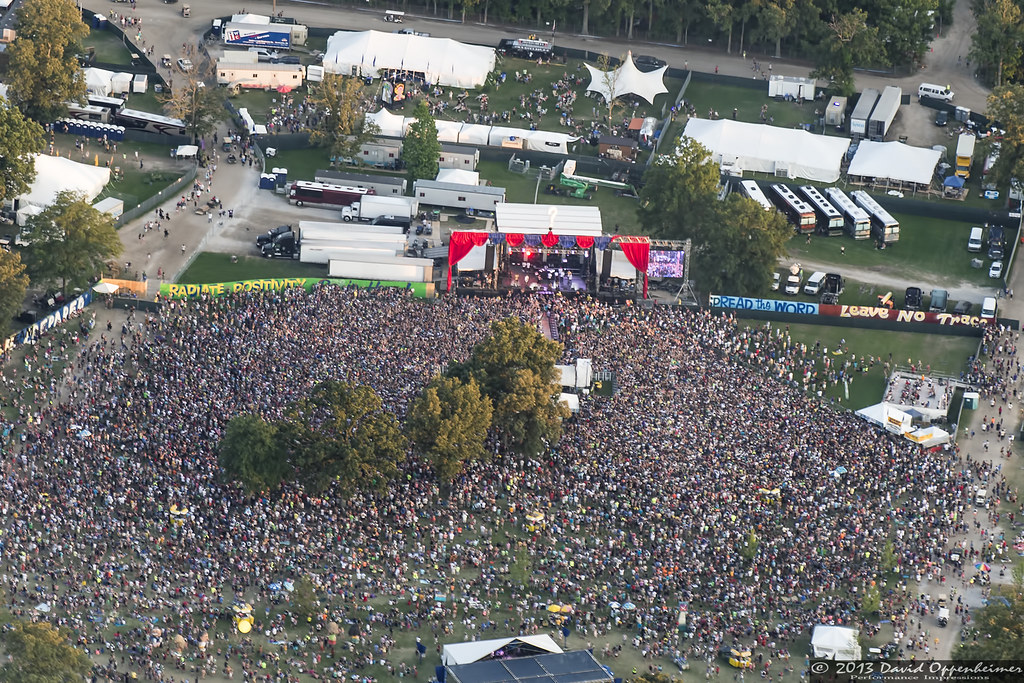This is an aerial photograph taken by David Oppenheimer capturing the 2013 Bonnaroo Music Festival in Tennessee. At the center of the image is a brightly lit festival stage adorned with red and blue drapes. A band performs under stage lights. Flanking the stage, there are banners with messages such as "Spread the Word, Leave No Trace" and "Radiate Positivity." A vast crowd fills the area, converging around a small copse of trees in the middle. Behind the stage, numerous 18-wheelers, tour buses, and tents are visible. Additionally, cranes, small trucks, and people moving to and from a parking lot can be seen. At the bottom of the photograph, the name "2013 David Oppenheimer" is inscribed. In the background, a roadway lined with trees completes the scene, emphasizing the festival's extensive layout.